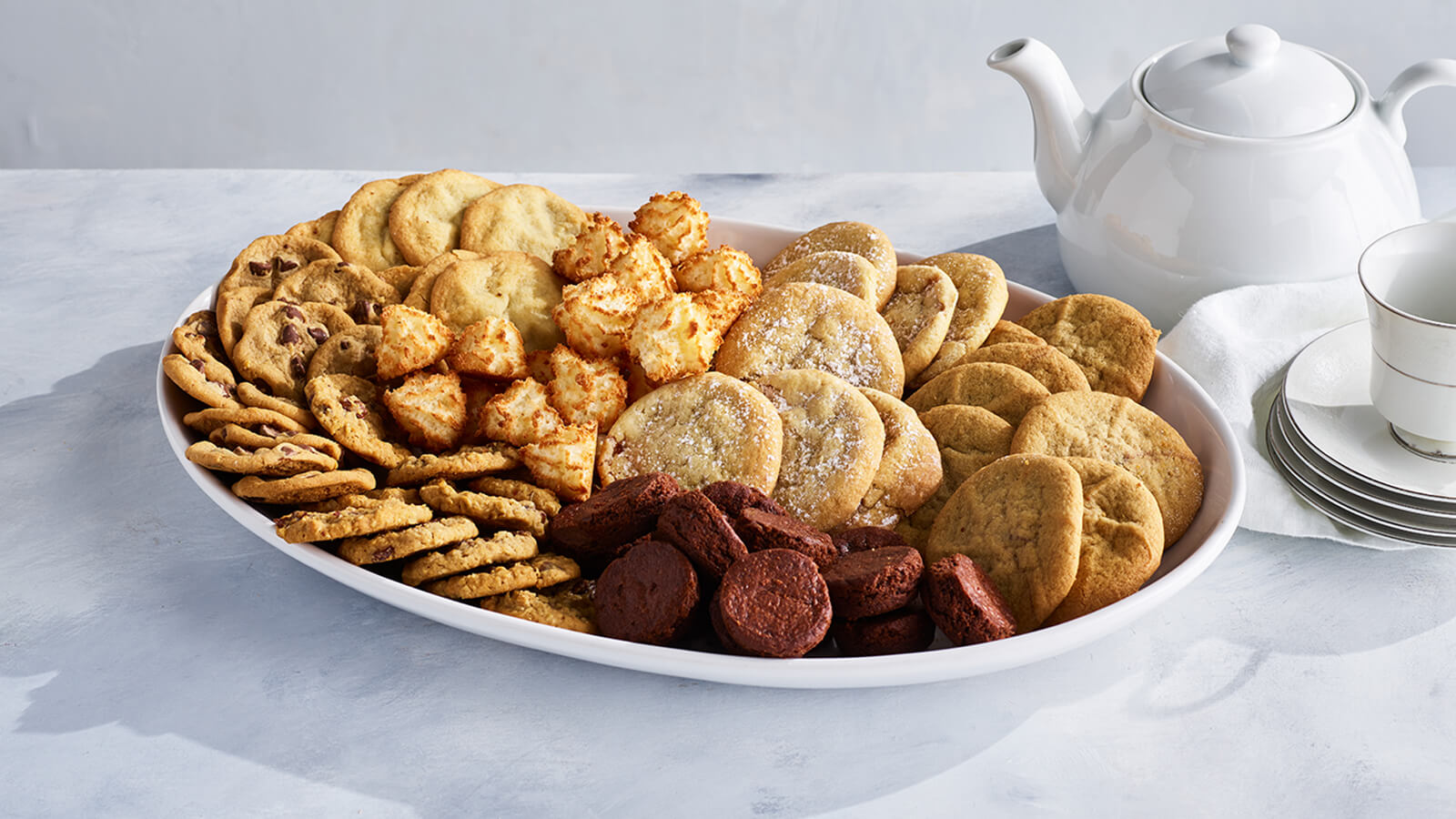In the photograph, a large white ceramic platter is elegantly arranged on a gray and white marble countertop, showcasing an assortment of cookies for what appears to be an event or party. The array of cookies includes chocolate chip cookies, sugar cookies, macaroons, snickerdoodles, peanut butter cookies, and round brownies, which contrast with the predominantly golden hues of the other cookies. The platter is flanked by a white teapot and a neatly stacked arrangement of four white saucers with a teacup on top, partially shielded by a white linen napkin. The teacup is distinguished by a silver rim and a silver band, which is echoed in the saucers. The minimalist background features a subtle sliver of a white wall, complementing the clean and monochromatic aesthetic of the scene, which is punctuated by the warm, inviting colors of the cookies.